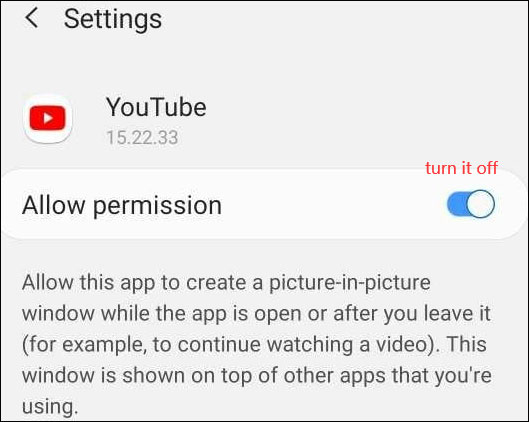This image, possibly captured from a smartphone or computer screen, displays the settings interface of an application. The background is a light gray, and at the top, there is a back arrow icon pointing to the left, next to the word "Settings" written in bold. Directly beneath this, there is a white circular icon featuring a red rectangle with a white play button in its center, denoting the YouTube app version 15.22.33.

Below the YouTube icon, there is a rectangular, white-edged button with rounded corners that says "Allow permission." At the end of this button, there is a blue slider bar with a white slider knob positioned to the far right, indicating that the permission is currently enabled. A small note in red text above this toggle reads, "Turn it off."

At the bottom of the interface, black text explains the purpose of this setting: "Allow this app to create a picture-in-picture window while the app is open or after you leave it (for example, to continue watching a video). This window is shown on top of other apps that you're using."